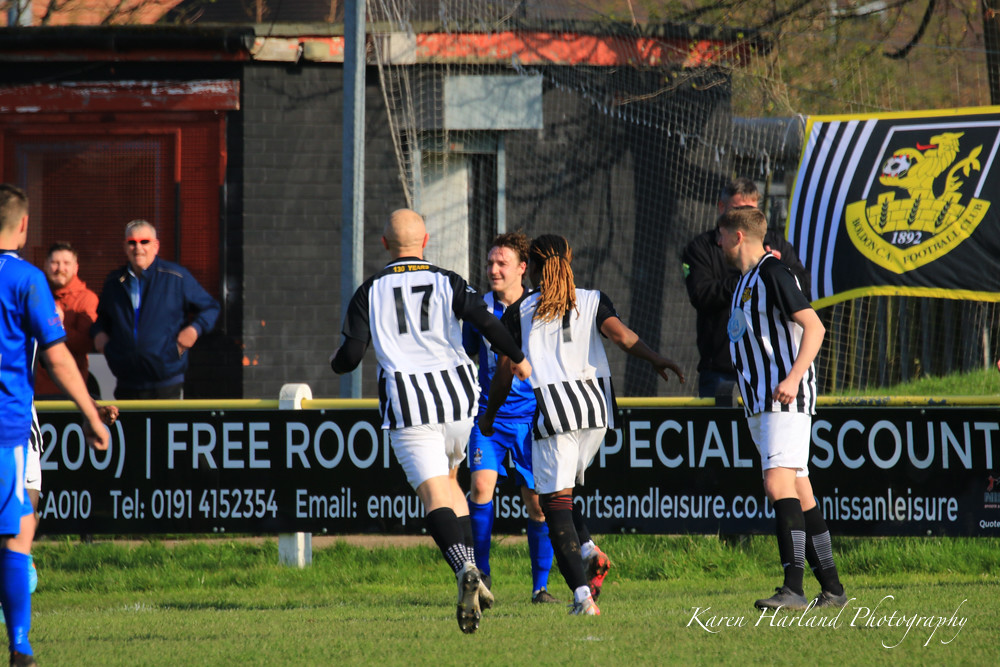This photograph captures an outdoor soccer game in action, featuring teams in distinctive uniforms: one team in black and white striped shirts with white shorts, and the opposing team in blue shirts, shorts, and socks. Prominently displayed on the metal fence behind the players are partially visible advertisements, including phrases like "Free Route," "Special Discount," and contact details such as "Telephone 0191-415-2354" and "Email queries at somethingsportslandsher.co.uk." The larger backdrop includes a gray brick building with a weathered roof and a net hanging from a pole. Spectators can be seen on the other side of the field. The players in motion include two individuals with the numbers 17 and 7 on their backs, alongside others, all engaged in the fast-paced action of the game. The bottom right corner of the image is marked with "Karen Harland Photography."